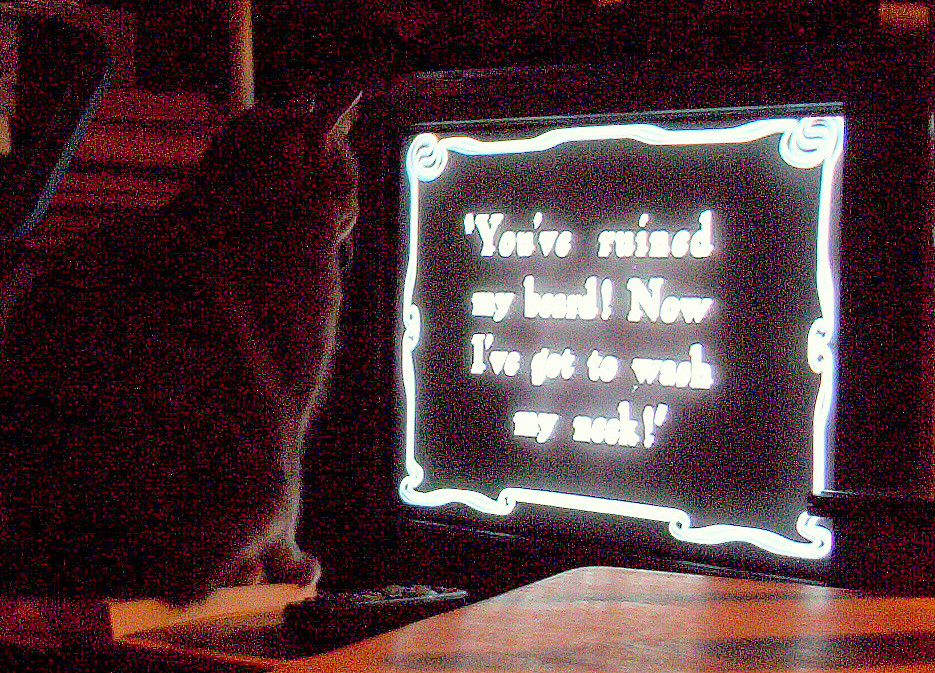The photo features a chubby cat sitting on the left side of a wooden table, fixated on a glowing display that appears to be a television screen. The image is grainy and slightly out of focus, adding to the sense of darkness enveloping the scene. The screen, which has a white border and white text on a black background, prominently displays the message: "You've ruined my beard! Now I've got to wash my neck!" The cat's gaze is intently locked onto the text, and next to the cat, a remote control can be seen. The overall setting suggests an indoor environment, with no other animals or significant objects visible.